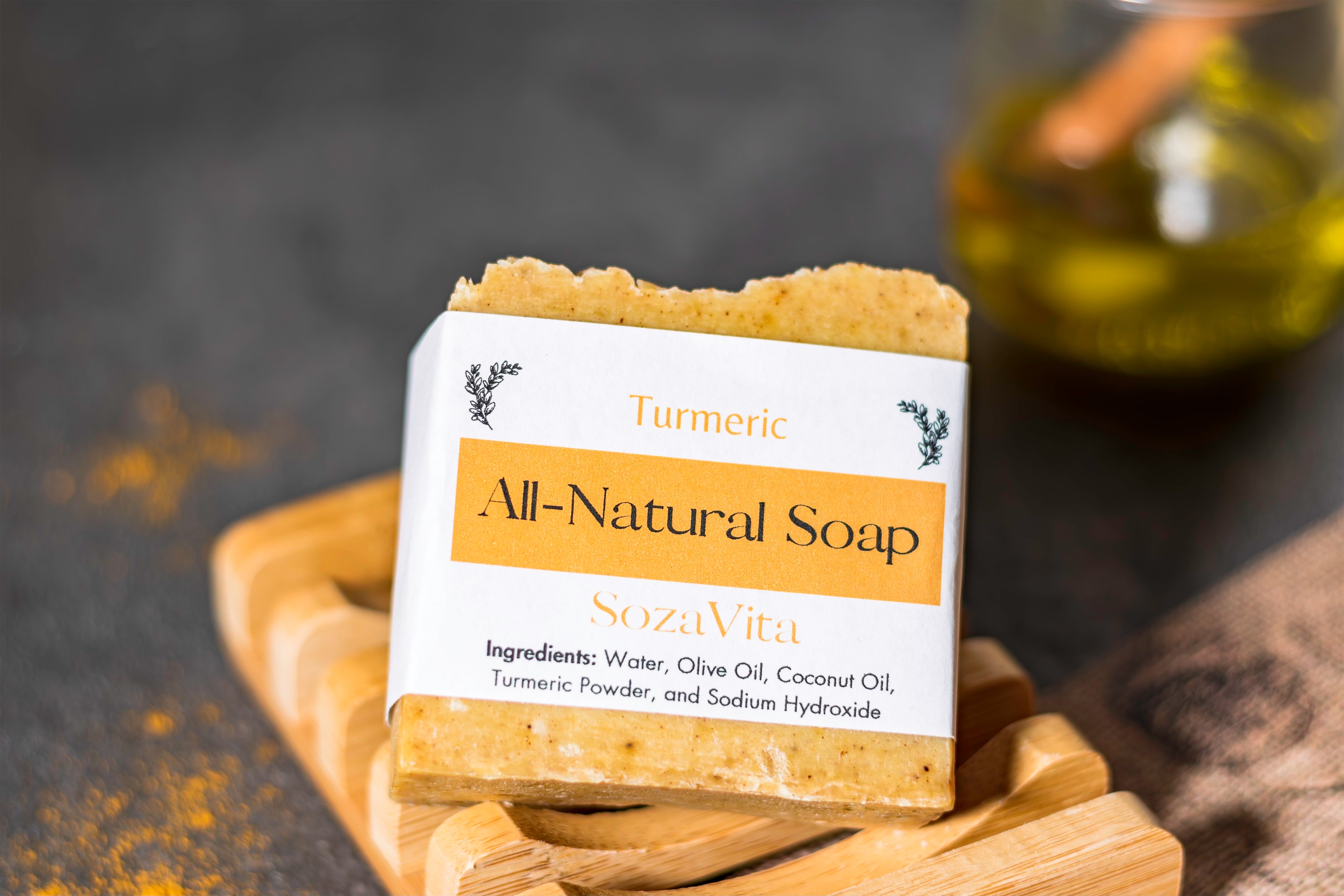In this close-up photograph, a bar of all-natural turmeric soap named "Sousa Vita" is prominently displayed on a wooden soap dish. The soap boasts a rich orange color speckled with brown and white flecks, likely from its natural ingredients. The soap's jagged top edge contrasts with its perfectly straight bottom, suggesting it was meticulously cut. It is encased in a white paper wrapper with a yellow banner that showcases bold black lettering reading "Turmeric All-Natural Soap." The brand name "Sousa Vita" is clearly printed below this banner, followed by a list of ingredients including water, olive oil, coconut oil, turmeric powder, and sodium hydroxide. The label also features two decorative etchings on its corners and a faint background image of olive oil. The soap sits atop a blue fabric mat, and the backdrop reveals a blurred black countertop with a glass vial of olive oil, some turmeric sprinkles, and a wooden stirring stick, adding a rustic charm to the scene.